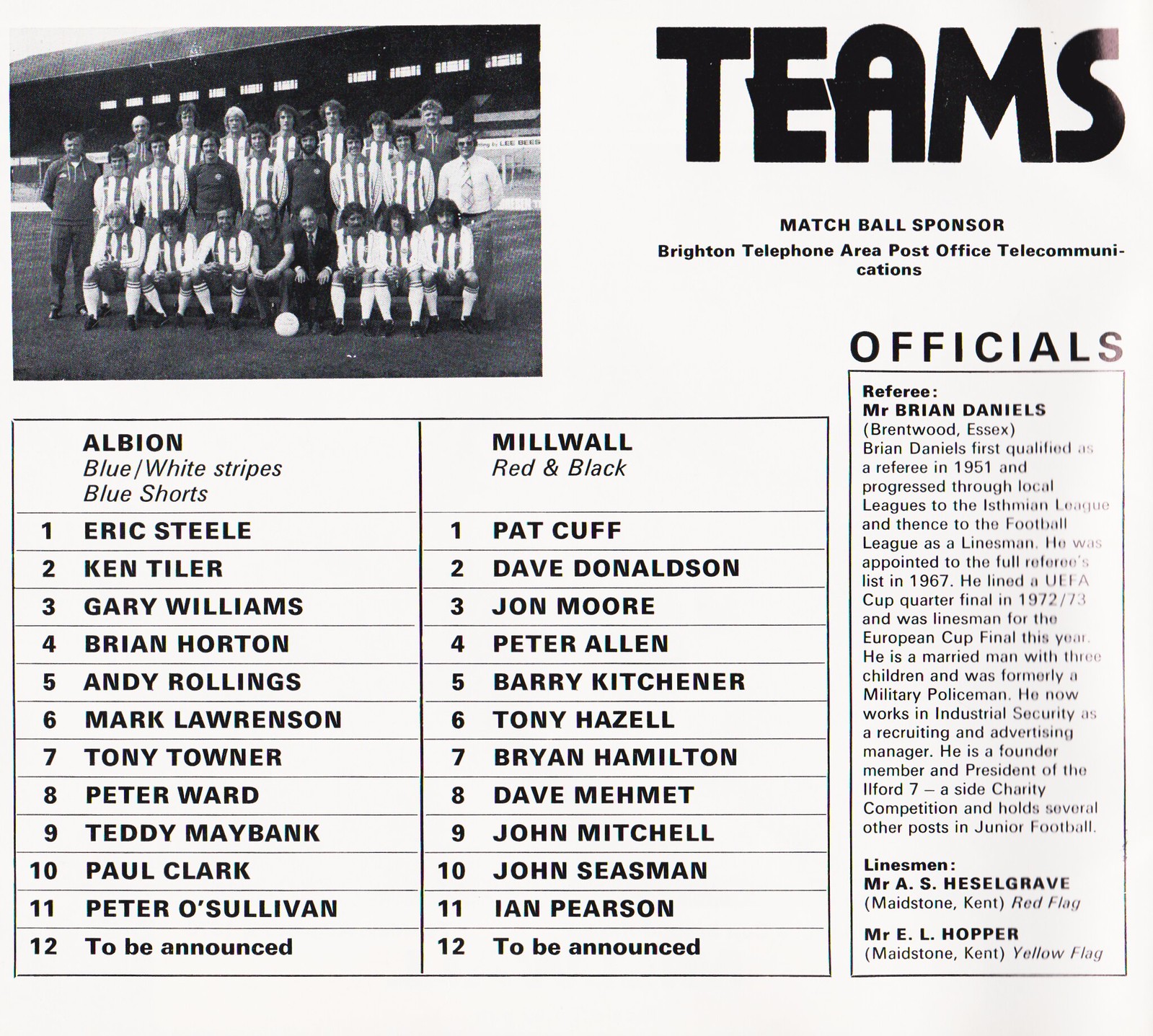This image is a black-and-white page from a soccer team program. The upper left corner features a black-and-white photograph of a soccer team posing on a field with a ball in front of them. The image has a white background with large black letters in the upper right corner reading "Teams," and the subtitle "Match Ball Sponsor, Brighton Telephone Area, Post Office Telecommunications."

The bottom portion of the page is divided into three columns. The left column lists the players for the team called Albion, featuring blue and white striped jerseys with blue shorts. The players listed are:
1. Eric Steele
2. Ken Tiger
3. Gary Williams
4. Brian Horton
5. Andy Rollings
6. Mark Lawrenson
7. Tony Towner
8. Peter Ward
9. Teddy Maybank
10. Paul Clark
11. Peter O'Sullivan
12. To be announced

The right column lists the players for Millwall, who wear red and black uniforms. The players listed are:
1. Pat Cuff
2. Dave Donaldson
3. John Moore
4. Peter Allen
5. Barry Kitchener
6. Tony Hazel
7. Brian Hamilton
8. Dave Mehmet
9. John Mitchell
10. John Seisman
11. Ian Pearson
12. To be announced

The center column is designated for the officials. The referee is Mr. Brian Daniels from Brentwood, Essex. His career highlights include qualifying as a referee in 1951, progressing through local leagues to the Eastman League, and later to the Football League as a linesman. He was appointed to the full referee list in 1967 and has significant experience, including lining a UEFA Cup quarterfinal in 1972-73 and being a linesman for the European Cup final this year. He is married with three children, a former military policeman, and currently works in industrial security as a recruiting and advertising manager. He is also a founder member and president of the Ilford Seven, a side charity competition, and holds several other posts in junior football. The linesmen are Mr. A.S. Hesselgrave from Maidstone, Kent (red flag), and Mr. E.L. Hopper from Maidstone, Kent (yellow flag).